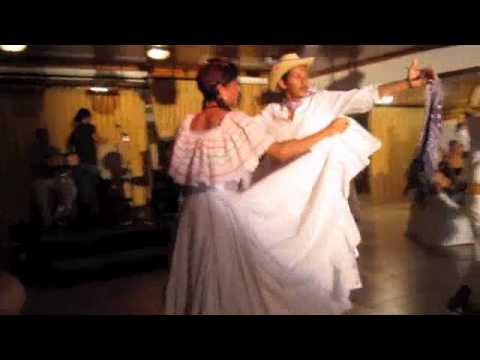The image is a full-color, square photograph taken indoors under artificial lighting, giving it a somewhat blurry appearance. It features a black horizontal border at the top and bottom, framing the scene. The main focus is a Hispanic couple dancing in traditional attire. The woman wears a long, light pink dress with ethnic designs and has her hair pulled back in a ponytail. The man is dressed in a white button-down shirt with the sleeves rolled up to his elbows and a straw cowboy hat. The couple is set against a backdrop where you can see a two-tiered black stage on the left, with a band playing under dim lighting. The band and their instruments are only partially visible, highlighted by overhead lights. Behind the couple, there's a dull yellow wall, and in the distance to the right, a group of people in white dresses can be observed. The wooden dance floor and the overall dim lighting add a nostalgic, almost cinematic feel to the scene, reminiscent of a scene taken from a film.